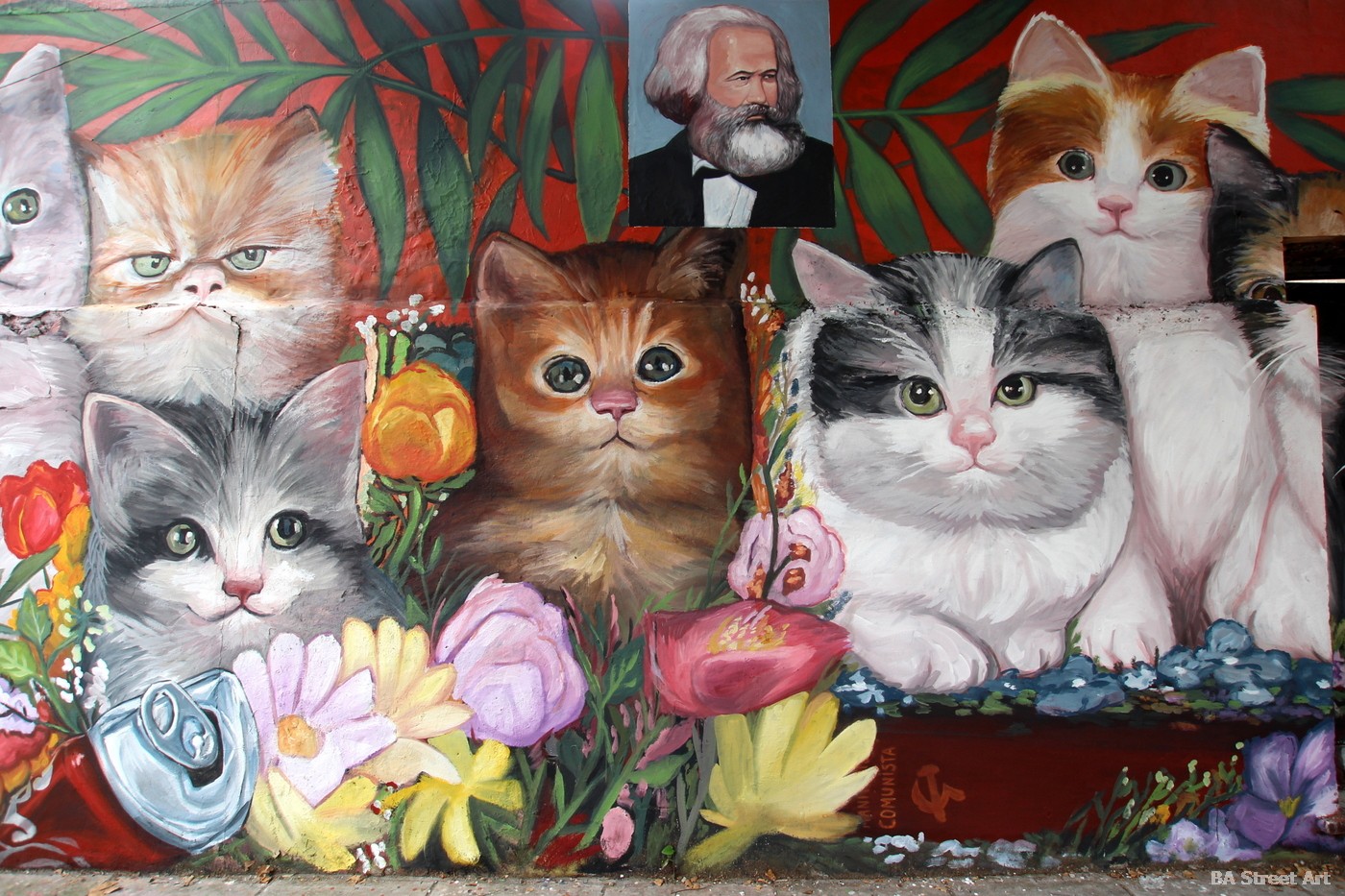The mural features a vividly detailed painting of seven small, adorable cats, each distinctly colored. From right to left, the cats are: a black and white cat, an orange and white cat, a gray and white cat, an orange tabby, another gray and white cat, a slightly grumpy-looking orange and white cat, and partially visible at the far left, a very light grayish-white cat. The background is predominantly red with green plants interspersed throughout, creating a lush and vibrant setting. At the forefront, there are colorful painted flowers in hues of white, yellow, purple, red, and orange. Additionally, a crushed Coca-Cola can can be seen near the bottom of the mural. The section of the mural where the cats sit also features a red book adorned with a hammer and sickle emblem, accompanied by the word "communista." Dominating the upper center of the mural is a portrait of Karl Marx, characterized by his large gray beard and fluffy hair, wearing a black suit and white shirt, and gazing towards the right.